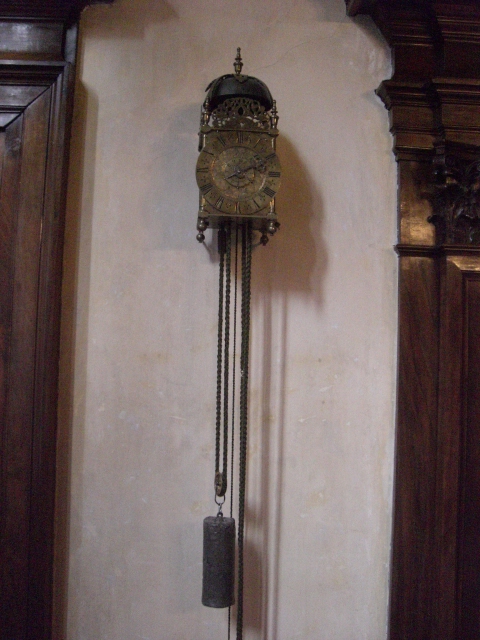A detailed caption for the given image could be:

"A beautifully aged clock hangs prominently on a wall, exuding an aura of antiquity and timelessness. This clock, though reminiscent of a traditional cuckoo clock, lacks the characteristic bird, making it a unique piece. The gold face of the clock is adorned with Roman numerals, standing out amidst the rich patina that envelops the entire piece, lending it an old-world charm. The clock features intricate chimes that hang gracefully down, with a large cylindrical charm on the right side adding to its distinct elegance. An ornate dome crowns the top of the clock, culminating in a delicate spire. The setting appears to be within a church, enhancing the clock's historical and reverent presence. The meticulous details of the timepiece, from its golden face to its patinaed surface, tell a story of a bygone era, preserved in the heart of this sacred space."